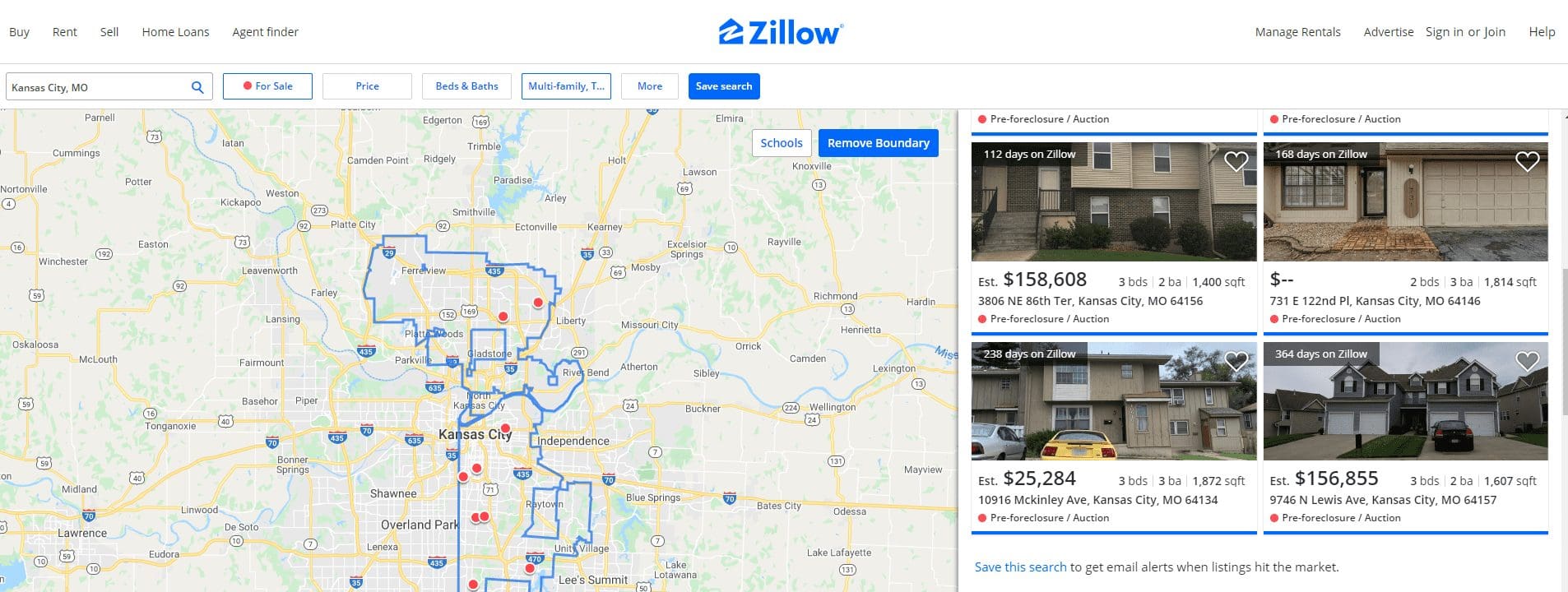A Zillow real estate search page displays various home listings in Kansas City, Missouri. The navigation bar at the top includes options to buy, rent, sell, access home loans, find an agent, and utilize the finder tool. The user is specifically searching for homes for sale, focusing on price, as well as the number of bedrooms and bathrooms, and potentially interested in multi-family units despite the text being small and difficult to read.

The map below highlights the central area of Kansas City, indicated by nine distinct red dots, each representing a house for sale. Four properties on the right side of the screen provide additional details such as listing dates and partial views of the homes. Of these, three are visibly two-story houses, while one lacks a complete view, making it unclear. The visible prices for three of the homes are $158,000, $25,000, and $156,000, while the price for the obscured property remains unspecified.